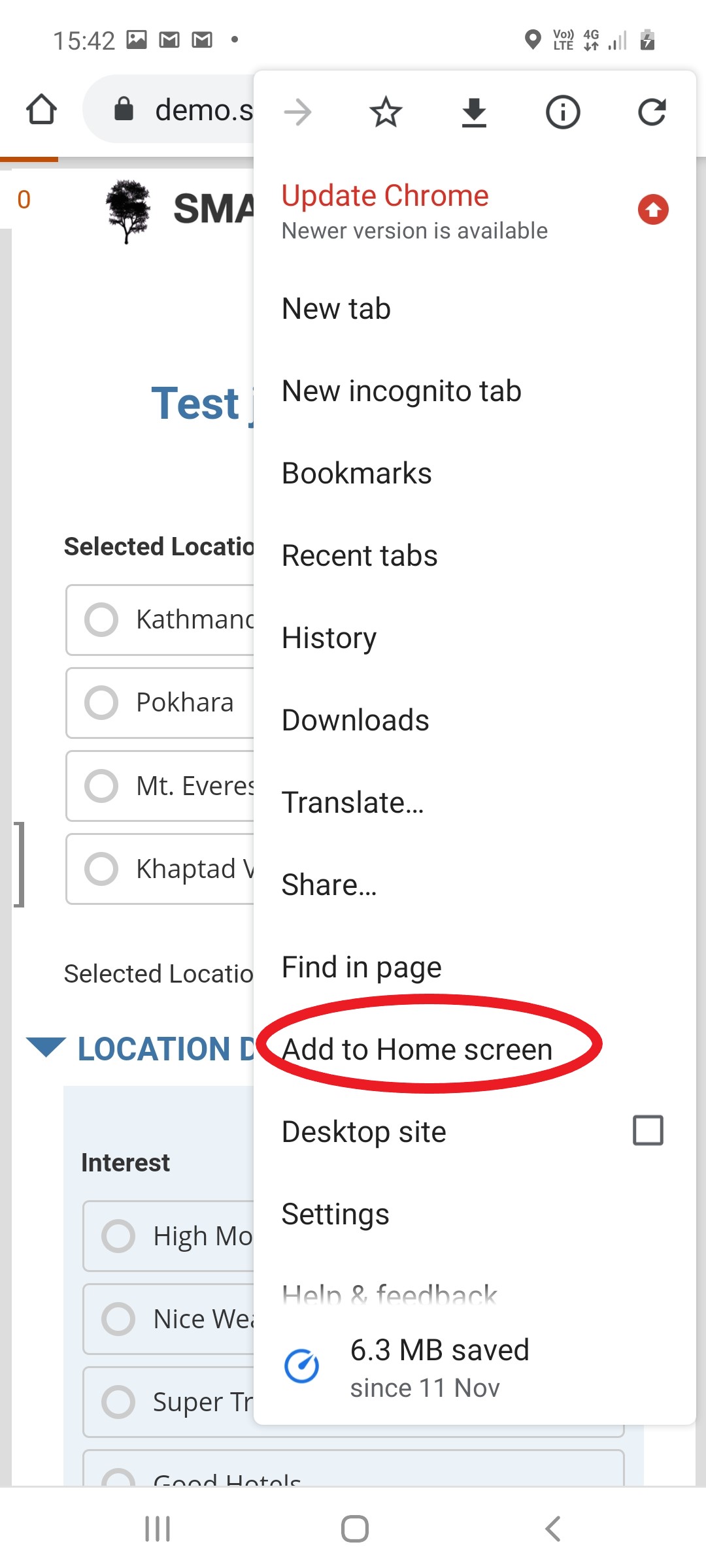In this image, the screen displays a web browser session, specifically in the Firefox browser, which is identifiable by its distinctive home icon. The address bar shows a partial URL that reads "demo.s," though it is partially obscured by another overlay. This overlay is a large dialogue box with the prominent header "Update Chrome" in dark red font. The dialogue box lists several browser options, including "New tab," "New incognito tab," "Bookmarks," "Recent tabs," "History," "Downloads," "Translate," "Share," "Find in page," and "Add to home screen," with the latter being highlighted by a red circle. Below that, additional options such as "Desktop site," "Settings," and a note indicating "6.3 megabytes saved since November 11th" are visible. In the background, barely discernible text mentions "task," "selected location," and various geographic names like "Kathmandu," "Pokhara," "Mount Everest," and "Captad." These background words appear to relate to different locations.